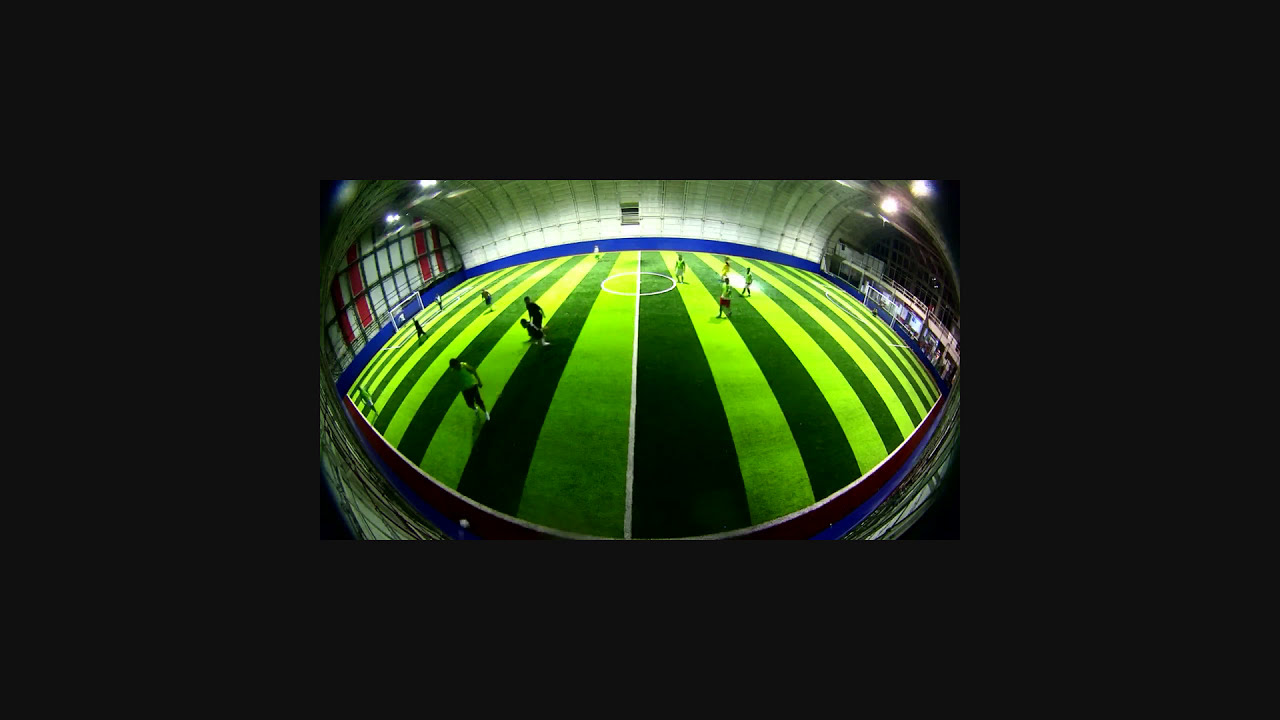The image captures an intense indoor soccer scrimmage between two teams, one in dark green uniforms and the other in light green uniforms. The field features an alternating pattern of dark green and light green stripes, giving it a visually distinctive appearance. At the center of the astroturf field is a white circle intersected by a white line stretching across it. The fisheye lens used to take the photo distorts the image, creating a spherical effect that makes the center appear closer while the edges seem to fade out. Players are scattered across the field, with some closer to the front on the left and others farther back, adding depth to the scene. The photo appears to be taken from an elevated vantage point, possibly the roof, and the black border framing the picture suggests a focused, framed view. The circular shape of the field and the arching walls in the background hint at an indoor facility specifically designed for soccer, adding to the immersive atmosphere of the game. There are no visible spectators, indicating that this could be a private practice match or an indoor league game with only the players present.